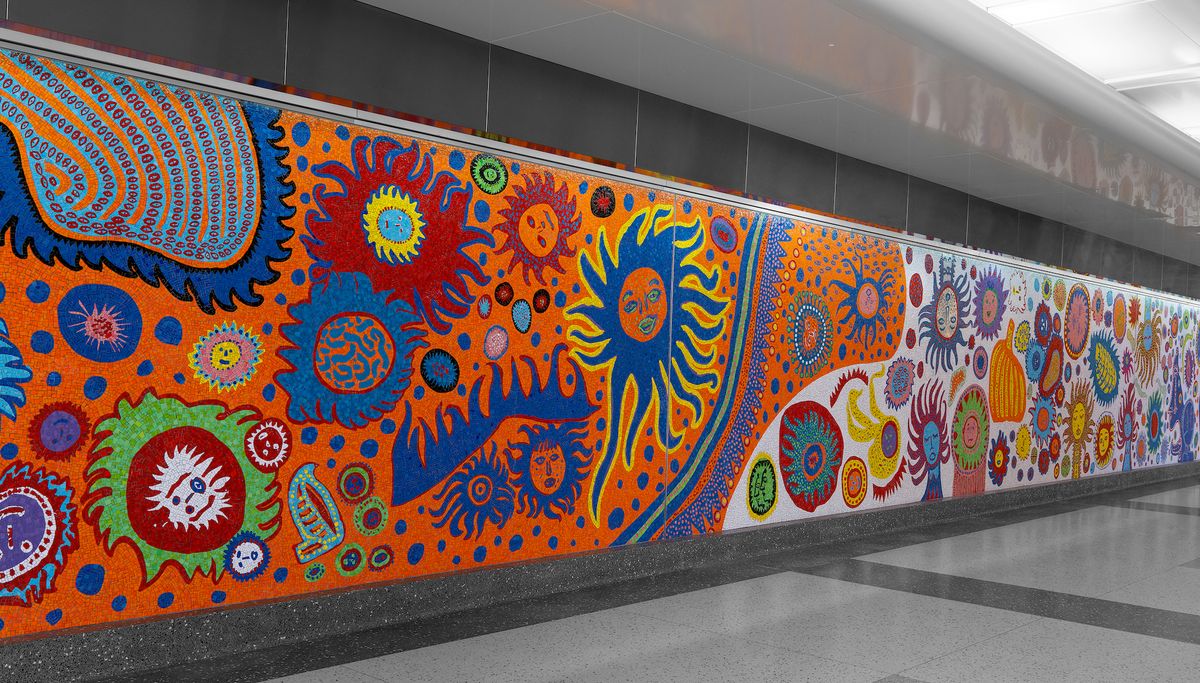This image showcases a vibrant and colorful abstract mural displayed on a wall within a brightly lit public or institutional space, notably enhanced by a polished linoleum or faux marble floor. The mural, which spans from left to right, features a striking juxtaposition of colors, transitioning from a bright orange background on the left to a white background on the right. The artwork is adorned with numerous sun-like figures, many of which are anthropomorphized with faces that include eyes, noses, and mouths, and their radiating flares artistically depicted like hair. This mural exudes a fluidity in its design, incorporating a myriad of hues such as oranges, yellows, blues, reds, pinks, purples, and greens. The orange section predominantly showcases suns with radiating waves and fewer faces, while the white section incorporates more facial elements. An underlying theme suggests a possible Mesoamerican influence, contributing to its overall bright and happy appearance. The mural's intricacy and vivid color palette transform the space into a dynamic visual experience.